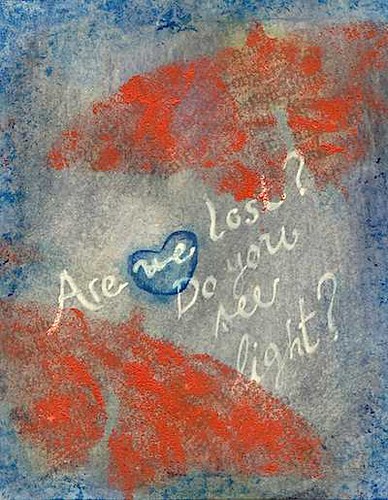This detailed, full-color image showcases a distressed painting style, prominently featuring shades of blue, black, white, yellow, and red. The textured background evokes a painted or chalk-drawn appearance, with notable blue undertones interspersed with white. Central to the artwork is a poignant message in a mix of printed and cursive text: "Are we lost? Do you see light?" Uniquely, the word "we" is encapsulated within a blue heart shape, though its intentionality is unclear. Adding to the complexity, the painting incorporates red and blue elements that resemble wings or feathers, extending to the sides, with the bottom part of the background appearing predominantly white.